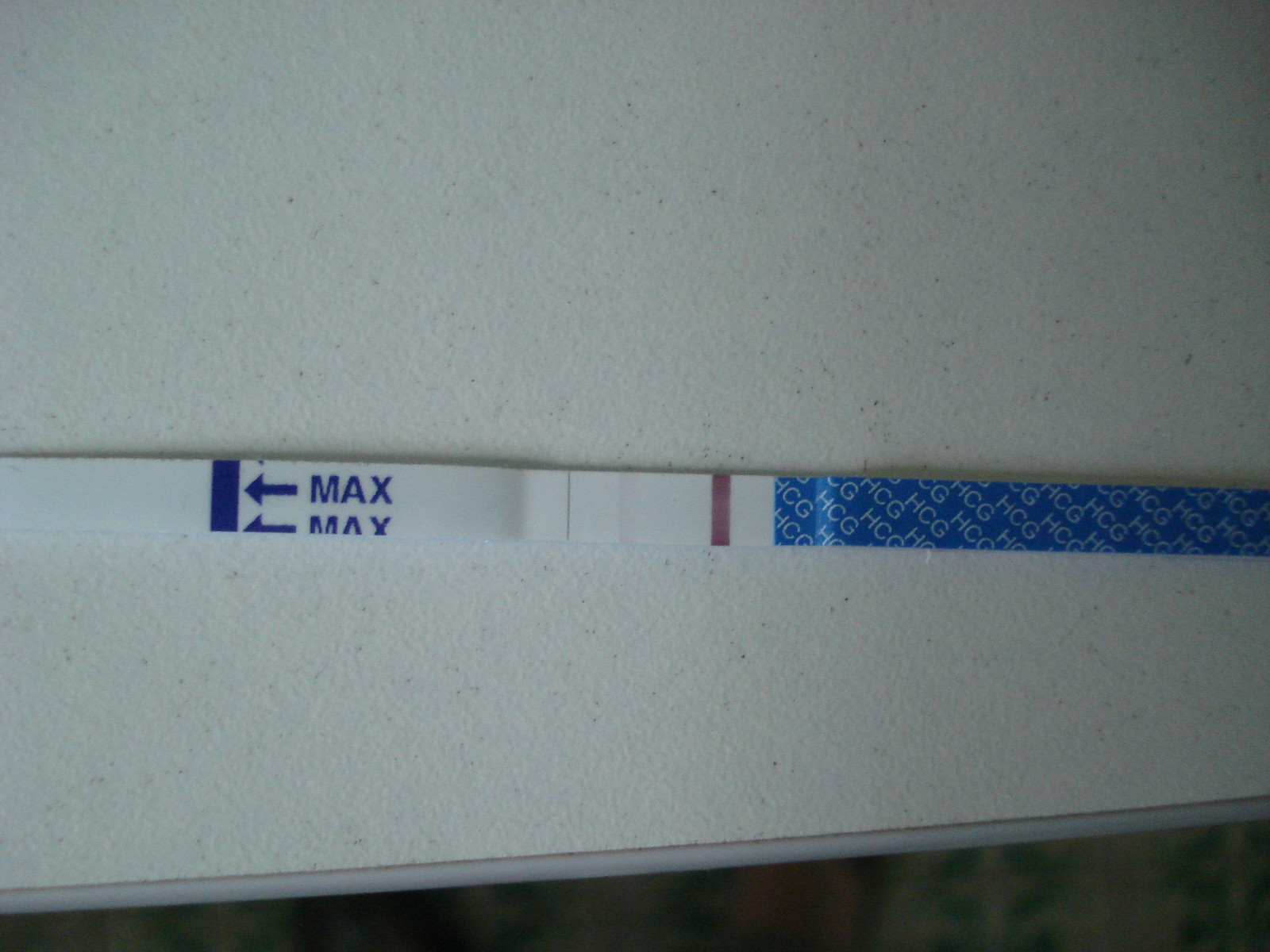A close-up image shows a strip of blue self-adhesive tape, intended for hanging lightweight items like posters on a wall. The protective paper backing is partially peeled off, revealing the sticky surface. White letters "HCG" are printed on the blue adhesive. The background appears to be a sturdy wall with a painted surface that might be speckled or made of another material. At the bottom of the image, there is a gray edge, which seems to be part of a doorway or wall trim, hinting at another room beyond. This area is out of focus but displays a mix of colors: gray, white, green, and various shades of brown. A noticeable symbol, a white plus sign within a green circle, is visible in the blurred background.